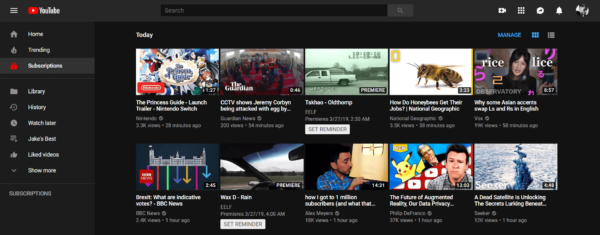The image depicts a YouTube homepage displayed in dark mode. The interface features a gray upper border and left-hand border with a black background behind the video thumbnails. In the upper left-hand corner, the classic red Play YouTube logo is positioned next to the word "YouTube." 

On the upper right-hand side, there are four icons: a grid icon for YouTube apps, a stream icon for YouTube Live, a notifications bell icon, and a profile icon. Centrally located towards the top is the search bar.

The left-hand sidebar includes various categories for navigation, including: Home, Trending, Subscriptions, Library, History, Watch Later, Jake's Best, Liked Videos, and a “Show More” option with additional subscriptions listed below.

The main content area is divided into two rows of videos, each containing five thumbnails. Above the video grid, a blue "Manage" button is situated in the upper right-hand corner. The visible video titles in the grid include:
1. The Princess Guide Launch Trailer - Nintendo Switch
2. CCTV Shows Jeremy Corbyn Being Attacked
3. Old Hump
4. How Do Honeybees Get Their Jobs? - National Geographic
5. Why Some Asian Accents Swap L's and R's in English
6. Brexit: What Are the Indicative Votes?
7. WAXD Rain
8. How I Got to 1 Million Subscribers
9. The Future of Augmented Reality
10. A Dead Satellite is Unlocking the Secrets Lying Beneath